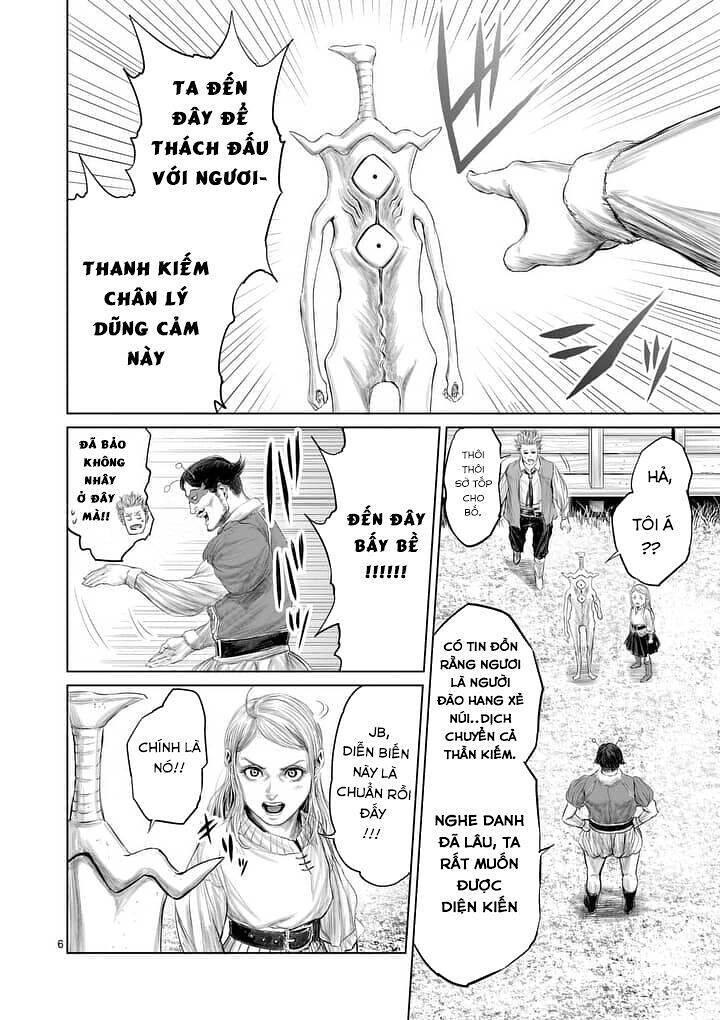The black-and-white comic book-style illustration is in portrait orientation and features a sequence of four panels, all in a foreign language that appears to be Vietnamese. The top panel is a large landscape scene depicting an unusual alien life-form without a head. The alien has two diamond-shaped eyes on its chest, a hairy midsection, skinny arms, and exposed upper hips. A person's hand with a long sleeve is pointing at this creature from the right side, with black hash marks accentuating the gesture.

Below this, on the left, are two smaller landscape panels stacked one above the other. The first of these shows a dark-haired man, possibly wearing a samurai outfit, featuring two antennas and a mask. He is engaged in conversation, pointing to the left with his left hand. The panel is filled with several speech balloons in the foreign language.

The panel beneath this depicts a young woman with light hair and eyes, facing the viewer. She is clad in a vintage-looking white blouse and appears to be engaging in dialogue, surrounded by multiple speech balloons in the foreign language. 

To the right of these two panels is a single, long portrait panel showing several figures interacting with the headless alien. Central among these figures is a person wearing a beige vest and black pants, standing over the creature, with speech balloons in foreign language on either side. Nearby, a young girl with a black skirt stands to the right of the creature, looking towards a man in the foreground wearing a dark gray shirt and balloon shorts, who has his back to the viewer. This panel also contains additional conversation balloons in the foreign language.

Overall, the page reflects a narrative involving humans and an alien entity, utilizing a detailed, sketch-like black-and-white artistic style.